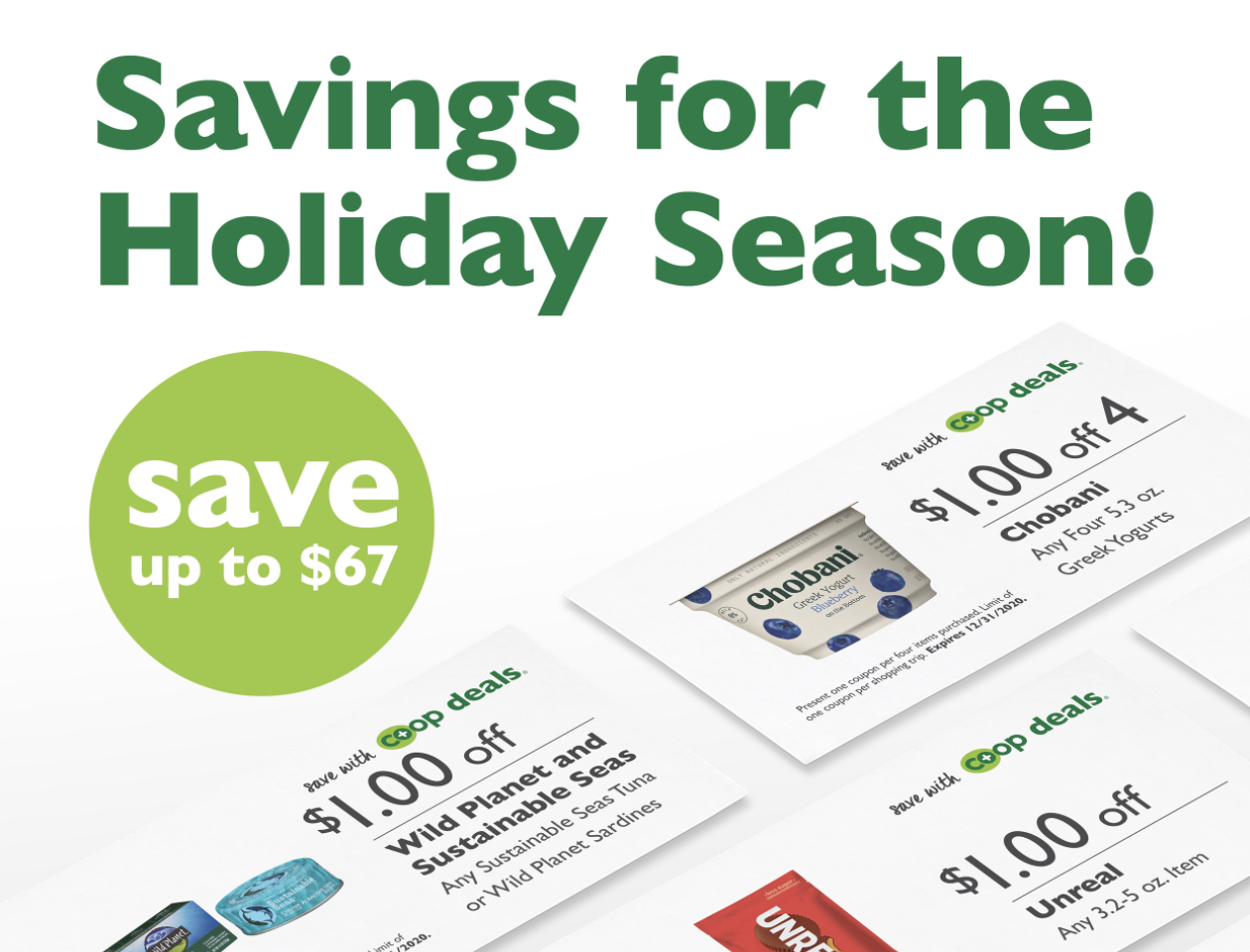On this page, we see an advertisement promoting savings for the holiday season. The phrase "Savings for the Holiday Season!" is prominently displayed in large, bold green font. Beneath it, there's a lighter green circle containing the text "Save up to $67." Additionally, the advertisement features three printed coupons:

1. The first coupon offers "$1 off" with Coop Deals on any Wild Planet or Sustainable Seas product, specifically sustainable seas tuna or Wild Planet sardines.
2. The second coupon provides "$1 off" with Coop Deals on any Chobani Greek yogurt (5.3 ounces). The coupon includes an image of a blueberry-flavored Chobani yogurt, adorned with blueberries.
3. The third coupon advertises "$1 off" with Coop Deals on any Unreal item (3.2 - 0.5 ounces). The coupon displays a partially visible, red Unreal bar.

Each coupon is designed to highlight the discount and the specific product in a visually appealing manner.